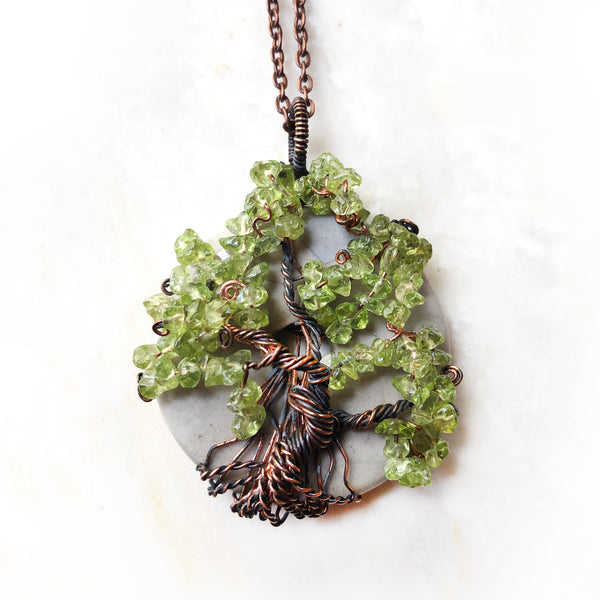This close-up photograph showcases a stunning pendant necklace, prominently positioned at the center. The pendant features a round, gray stone with a central hole, meticulously encased in intricately wrapped dark copper and black wires. These wires form an artistic depiction of a tree, with the trunk and branches extending gracefully around the stone. The tree’s leaves are represented by vibrant green peridot crystals, which are variably shaped into nuggets and chips. These green crystals add a lively contrast to the darker tones of the wires. The pendant, hanging from a rust-gold copper chain that runs vertically through the image, exudes a natural, earthy beauty. The overall design evokes a harmonious blend of nature and craftsmanship, highlighted by the intricate interplay of copper wiring and green gemstone leaves. There is no accompanying text or additional imagery, ensuring full attention to the pendant's exquisite details.